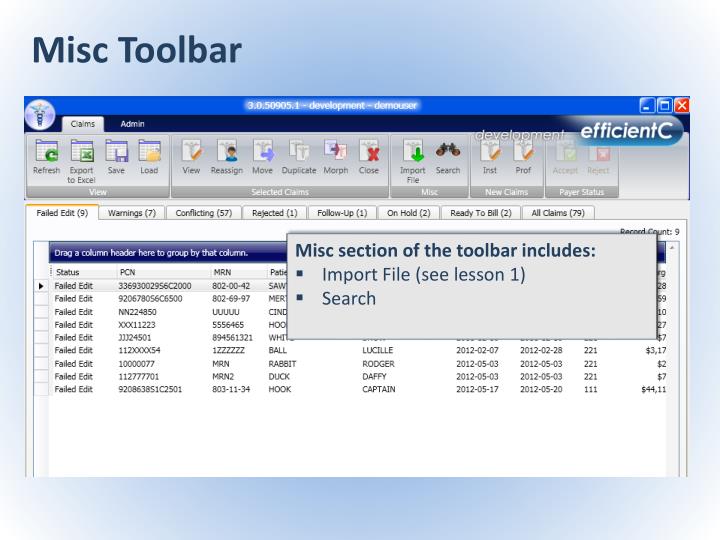The image showcases a screenshot of a computer application, likely a filing or financial software, titled "MISC Toolbar," with the program version "3.0.5.50905.1-development-demouser" displayed at the top. The interface, bordered by a light blue gradient, features a main toolbar with tabs such as "Claims" and "Admin." Under the "Claims" tab, there are four sub-tabs labeled "Refreshed," "Export to Excel," "Save," and "Load." Additional tabs to the right include functionalities like "Close," "Morph," "Duplicate," "Import," and "Search." Below these tabs, a list of files is shown, all marked with the status "Failed Edit." Superimposed on the image is a faint blue box listing the features of the MISC toolbar, including bullet points for "Import File, see Lesson 1" and "Search." A watermark reading "development efficiency" can also be seen over the image.